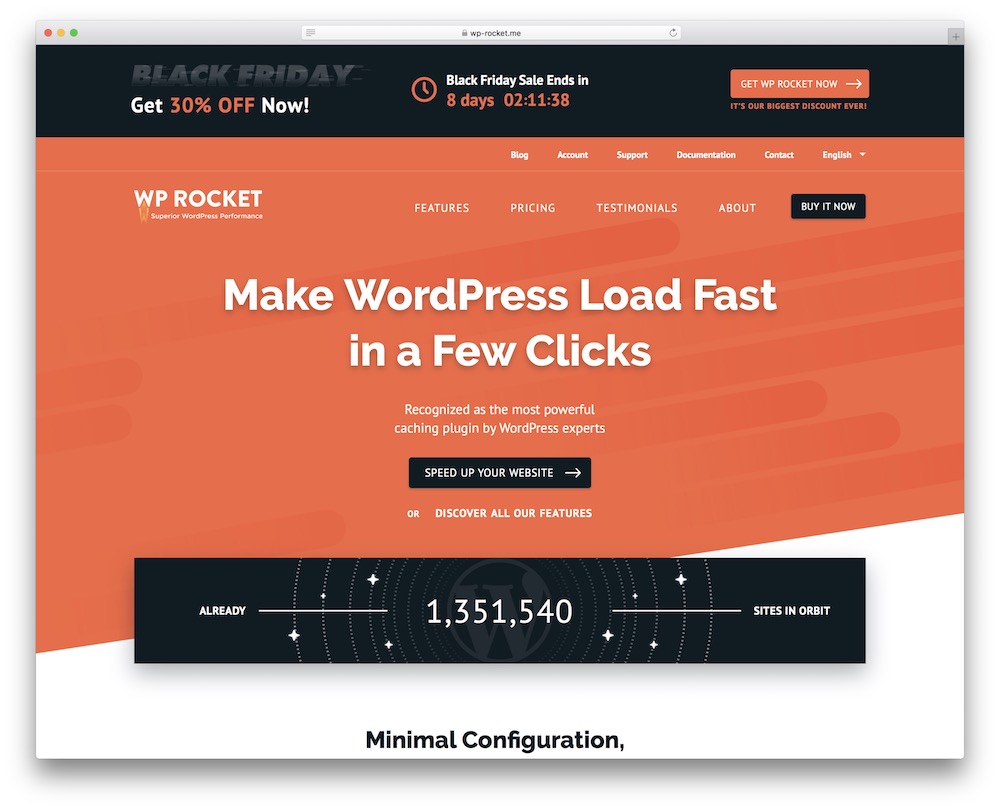A screenshot of a web browser displaying a Black Friday promotion for WP Rocket, a well-known caching plugin for WordPress. The advertisement highlights a 30% discount on the product, with the sale ending in eight days. The WP Rocket logo is visible, set against a simple background featuring orange, black, and white colors. The promotion emphasizes WP Rocket’s capability to significantly speed up WordPress websites with just a few clicks, touting its recognition as a powerful tool among WordPress experts.